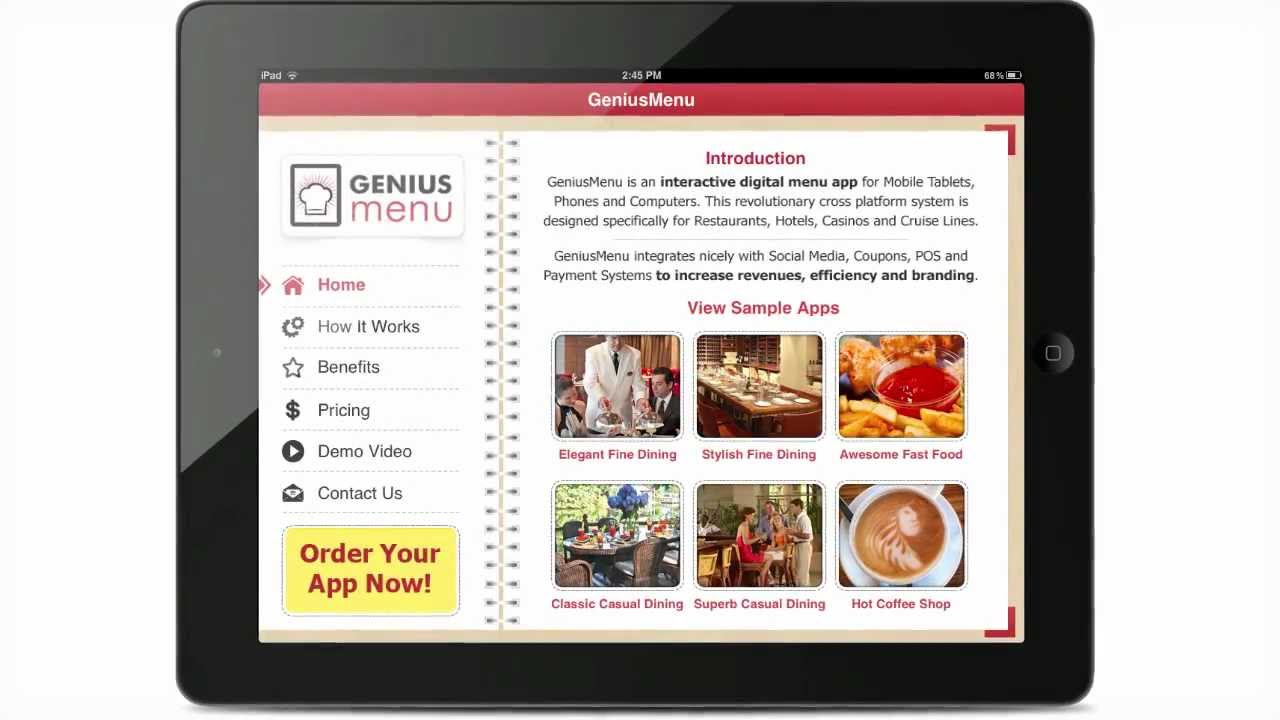In this image, we are looking at a digital display, likely on an iPad or a similar tablet, showcasing the Genius Menu. The screen appears to be split into two sections, resembling a binder or spiral menu, with the left portion displaying a third of a page. At the top of the left section, "Genius Menu" is prominently displayed, accompanied by a small chef’s hat icon. Below this title, there are several menu options listed in rows: Home, How It Works, Benefits, Pricing, Demo Video, Contact Us, and a bold red "Order Your App Now" button on a yellow-clicking sign. 

On the right side of the screen, there is an introduction to Genius Menu, describing it as an interactive digital menu app designed for mobile tablets, phones, and computers. This revolutionary cross-platform system caters specifically to restaurants, hotels, casinos, and cruise lines. It further explains that Genius Menu integrates seamlessly with social media, coupons, POS (point-of-sale), and payment systems to increase revenue, efficiency, and branding.

Beneath the introduction, there are six small images showcasing different dining scenarios: people sitting in a restaurant, a dining table set with formal dishware, French fries with ketchup, a fancy dinette in an outdoor setting, a casual dining experience, and a hot cup of coffee in a white cup. Additionally, there are clickable options labeled as "View Sample Apps," featuring categories like Elegant Fine Dining, Awesome Fast Food, and Hot Coffee Shop, illustrating the variety of digital menu styles available.